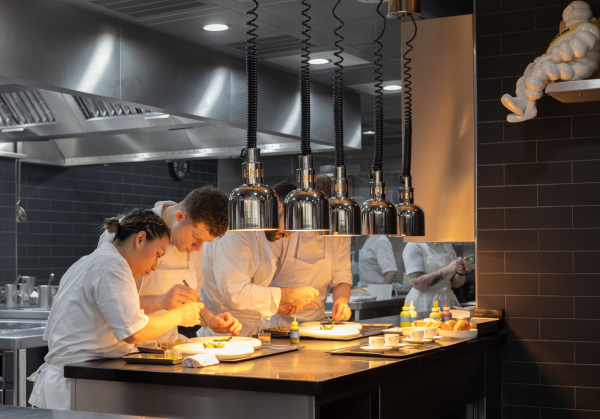The photograph captures a bustling restaurant kitchen scene indoors. The centerpiece is a large counter where a dedicated team of line chefs, dressed uniformly in white shirts and aprons, meticulously prepare dishes. Their focus is highlighted by an array of hanging pendant lights with coil cords, illuminating the counter. Small condiment bottles, resembling miniature mustard bottles, are neatly lined up next to them. 

In the foreground, a chef with dark hair tied in a bun and possibly wearing a hairnet, reaches across the counter, her right hand in motion. Next to her, another chef with short brown hair is bent over, concentrating on a task with a tool in hand. Further along the counter, partially obstructed by the pendant lights, are two more chefs engaged in their culinary work, their heads cut off in the image.

The background reveals more chefs, busily working on metal tables equipped with pots, pans, and a hanging ladle. Above them, metallic vents line the ceiling, maintaining the kitchen's airflow. 

A brown brick wall runs along the right side of the photograph, topped with a small white ledge in the upper right corner. Perched on this ledge is a noticeable figure—a little statue of the Michelin Man—observing the scene. The intricate details of this kitchen, from the reflective chrome fixtures to the lively orchestration of the chefs, paint a vivid picture of a high-paced, professional culinary environment.